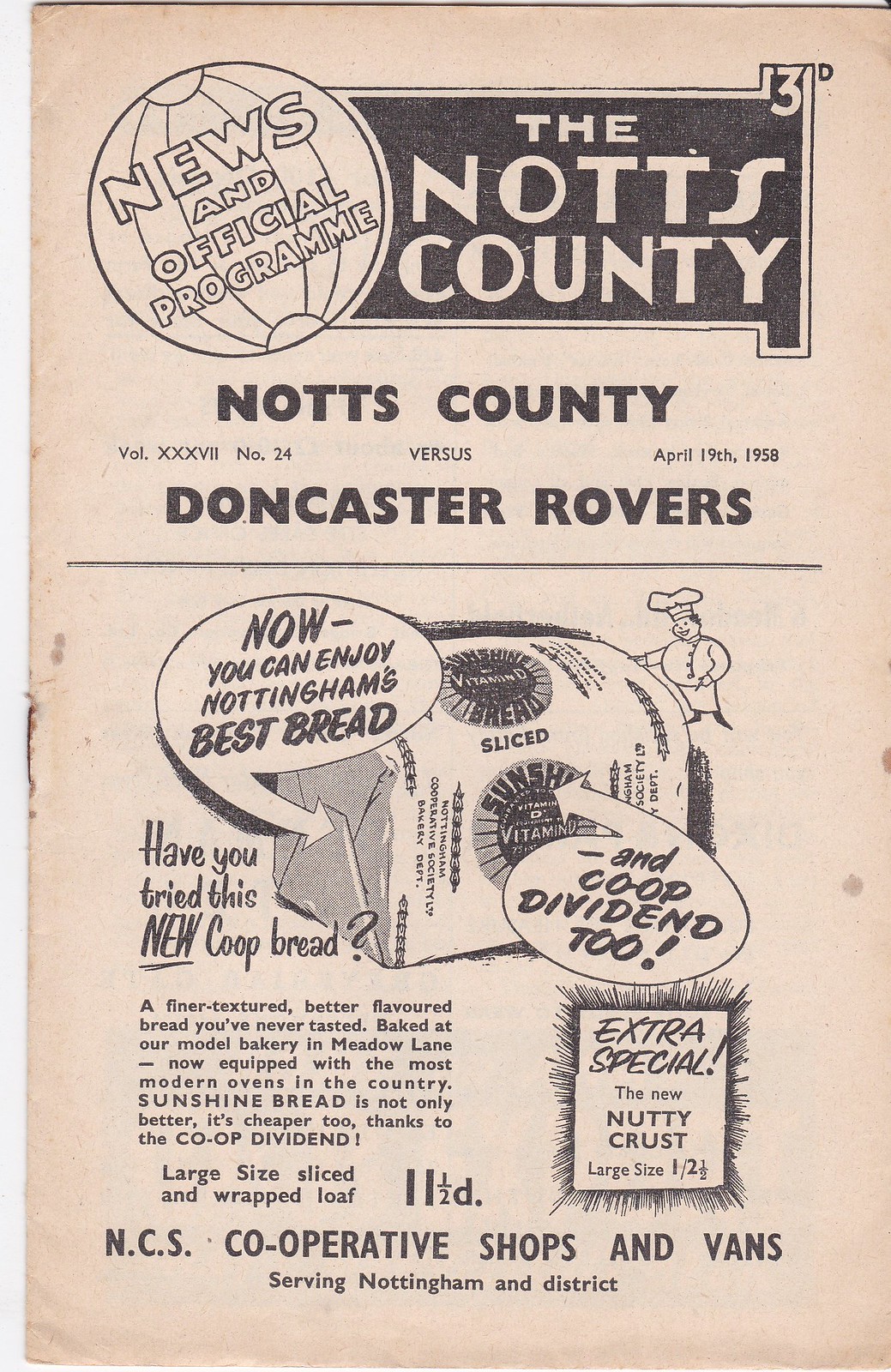This is a detailed description of an old black and white advertisement from April 19th, 1958. It appears to be a page from a newspaper or magazine. In the upper section, there is a large tilted globe illustration with "News and Official Program" written to its right, all set against a black background. To the right of this, there's a black banner that reads "Knotts County" with the number three in the upper right corner. Below this, in smaller black text, it states "Vol XXXVII, Number 24" and mentions the Doncaster Rovers match. 

Further down, there’s a prominent advertisement for bread featuring a 1950s-style loaf with a cheerful chef floating beside it, holding a chat bubble that says, "Now you can enjoy Nottingham's best bread." Another bubble to the right states, "And co-op dividend too." Beneath this chef, in vintage text blocks, it reads, "Have you tried this new co-op bread?" followed by a descriptive paragraph extolling the virtues of the bread, including its finer texture and better flavor. The ad assures customers that the bread is baked at their modernized home bakery on Meadow Lane and is cheaper due to the co-op dividend.

The ad continues with labeling the bread as "extra special," promoting their new nutty crust large loaf, priced at 11.5D. At the bottom of the page, it is noted that the NCS Cooperative Shops and Vans serve this bread throughout Nottingham and the surrounding districts. The entire page has a faded, pinkish newspaper tint, adding to its vintage appeal.